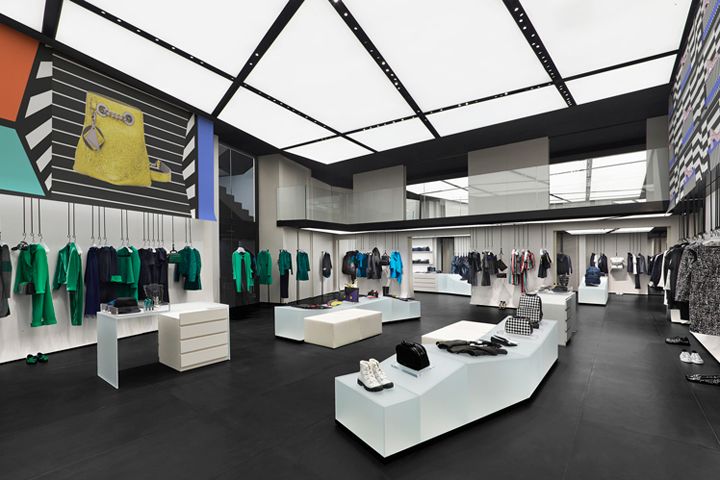This detailed photograph captures the interior of an upscale, minimalist clothing store. The store is encased in a tall, spacious, and modernistic design. The floor is a solid black slate, providing a stark contrast to the bright white ceiling, which is interspersed with black lines and dotted patterns, possibly designed to mimic a grid or mesh structure. The ceiling appears to filter natural light, potentially through smoked glass or other translucent materials.

The store's walls are mostly white, accented with geometric murals that incorporate black and white stripes, along with colorful elements such as orange, teal, purple, and yellow. Prominently on the left wall, a mural features a large yellow purse with a chain handle against a black and white striped background. Another mural on the back right wall displays geometric shapes in black, white, gray, and purple.

Clothing is strategically displayed in sparse, non-cluttered arrangements along the perimeter. On the left wall, green outfits, such as tuxedos and blazers, dominate. The back wall on the right holds attire in blue, black, and gray hues. No multiple sizes of the same garment are visible; instead, each piece appears to be unique and singularly hung, suggesting a high-end or custom-made approach.

In the center of the store are sleek white display tables and stands showcasing a selection of black and white accessories, which include patterned and solid shoes, purses, boots, a backpack, and handbags. The black and white checkered designs on some of the accessories stand out prominently.

There are no people present in the image, further emphasizing the clean, sophisticated, and exclusive ambiance of the store. The overall aesthetic is one of modern luxury, with geometric art and thoughtfully arranged clothing and accessories combining to create an elegant shopping environment.